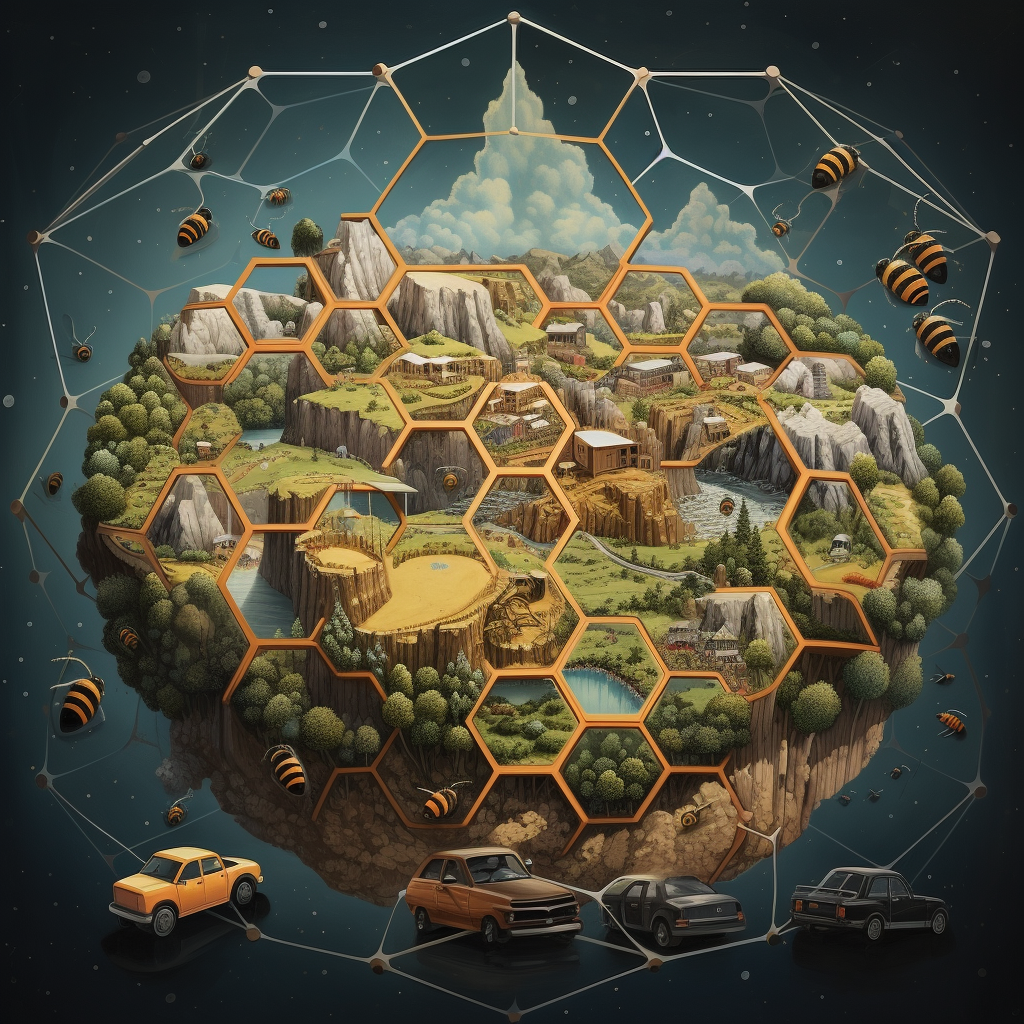The image is a striking piece of digital art that portrays a landmass floating in space, showcasing a diverse range of land formations including water bodies, grassy fields, and large rocky cliffs. The outer edge of the landmass reveals a cross-sectional view of the earth's dirt and crust, adorned with trees and rock fence borders. The scene is defined by a giant honeycomb structure hovering over the land, with enormous bees, some as large as vehicles, flying around. Stars twinkle in the background adding to the ethereal, otherworldly atmosphere. The bees, central to the artwork's theme, appear to be symbolically significant, as if emphasizing their crucial role in the ecosystem. The image intricately combines elements of nature and space, creating a surreal, almost dreamlike landscape divided into various segments reminiscent of a beehive.